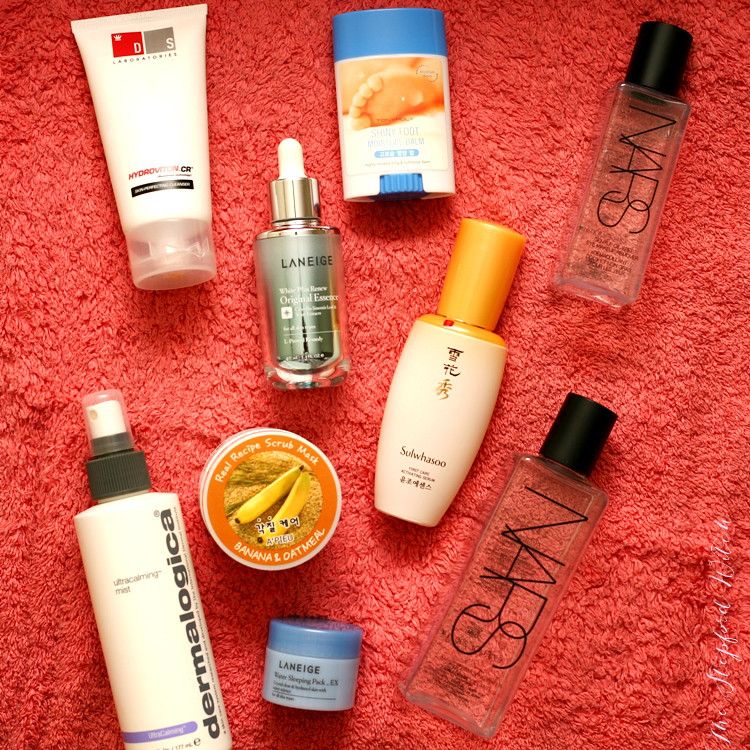On a vibrant pinkish-red fuzzy towel, a diverse array of makeup and skincare products are meticulously arranged. In the bottom right corner, the phrase "The Stepford Witch" is inscribed in an elegant, white cursive font.

**Right Side:**
- Two identical elongated clear bottles with black lids, labeled "NARS" in bold black font, resembling oversized nail polish bottles. The ingredients and size details are indiscernible.

**Left Side:**
- A white bottle, somewhat tubular but stout, possibly lotion, bearing the label "DS" with the "D" in a red square and the "S" in a gray square, followed by "Hydrovitron CR." The letters are clear, but the full label is not completely readable.
- Adjacent is a spray bottle with a white nozzle and a black lid, labeled "Dermalogica UltraCalming Mist," known for soothing skin, about the size of a standard perfume bottle.

**Middle:**
- A small travel-sized product resembling deodorant, labeled "Shiny Foot Moisture Balm," featuring an illustration of a white foot, with additional text in Japanese. The lid and twisting component of this balm are blue.
- An eyedropper bottle with a white nozzle, silver lid, and clear body, inscribed with "Laneige White Plum Renew Original Essence," though the print is fine and somewhat blurred.
- Beside it, a suntan lotion-shaped bottle with a pale orange lid and a white body, labeled "Sulwhasoo First Care," with accompanying Japanese writing.
- A small tin of "Real Recipe Scrub Mask, Banana and Oatmeal," its outer rim accented in orange and featuring images of bananas with Japanese script.

**Bottom:**
- A sophisticated silverish-blue container marked "Laneige Water Sleeping Pack EX," adding a touch of luxury and intrigue.

This impressive collection predominantly features travel-sized skincare products, offering a glimpse into an assortment of premium beauty treatments designed for various skin needs.